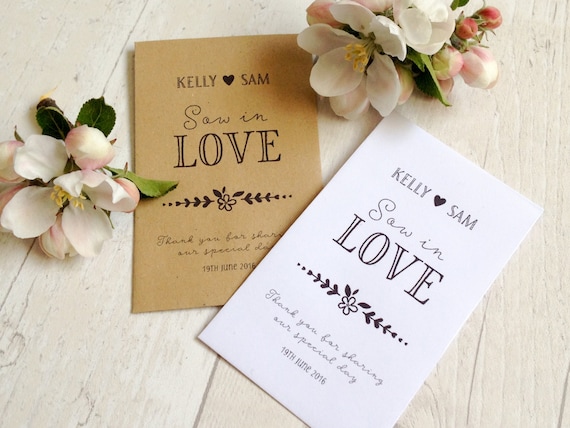The image depicts two wedding invitations placed on a light cream-colored wooden table with angled wood slats. The left invitation is brown, and the right one is white, both featuring identical black text. The text includes "Kelly ♥ Sam" followed by "so in love" in a cursive script, with a vine and flower decoration underneath. Below the decoration, the text reads "Thank you for sharing our special day, 19th June 2016." Overlapping the lower right corner of the brown invitation is the white invitation. In the upper section of the image, there are pink and white flowers with green leaves; a single flower appears to the left of the brown invitation, while a cluster of flowers is arranged above the invitations. The photograph is taken from above, indoors, and measures approximately four inches wide by three inches high.